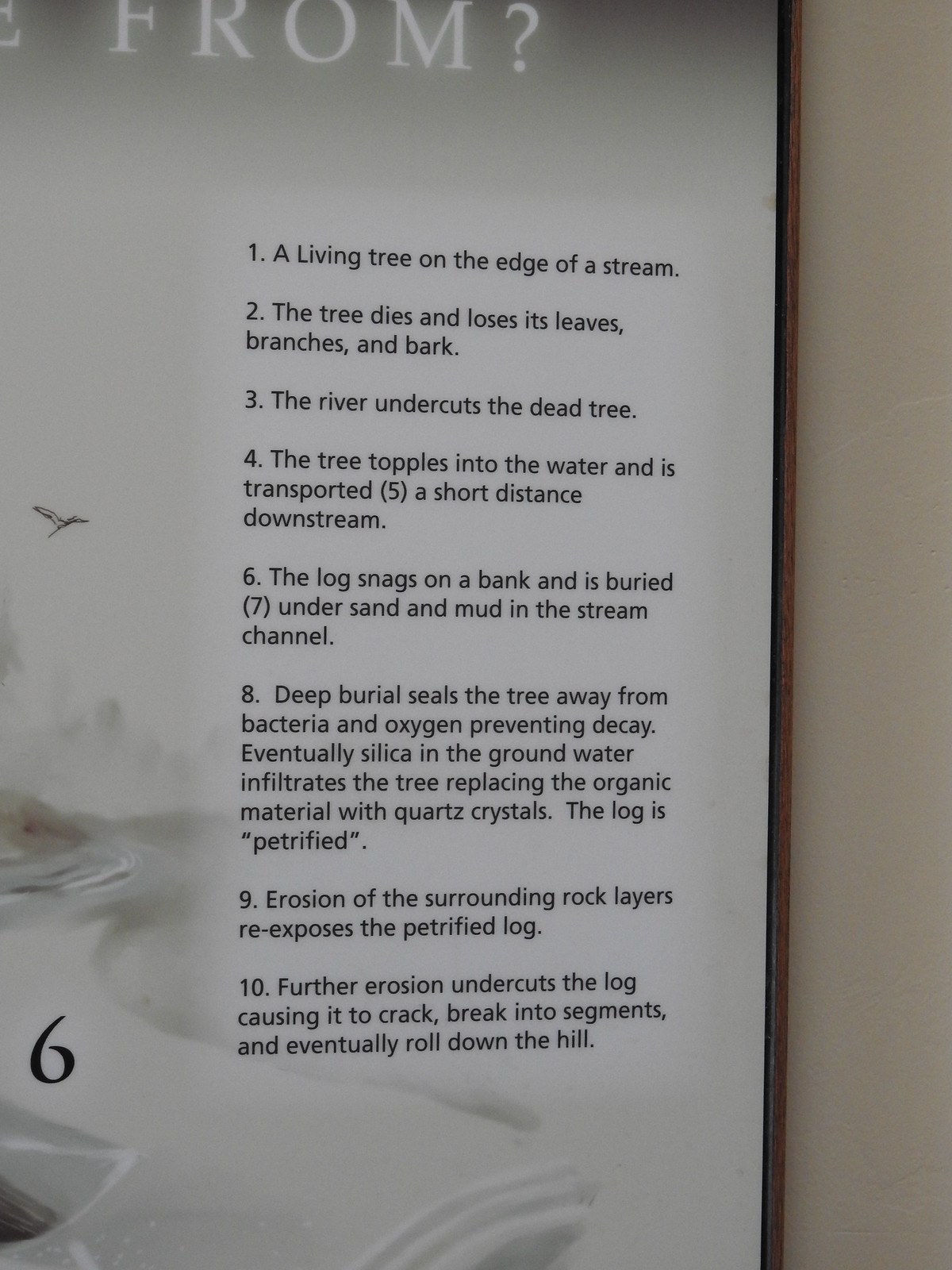The image features a close-up view of a page or poster measuring approximately six inches high by four inches wide, emphasizing the right edge. At the very top, printed in white with a question mark, is the phrase "word from?" which has a slightly ethereal appearance due to a white glow surrounding the text. Below this, a bulleted list numbered from one to ten narrates the life cycle of a tree. 

The list begins with "A living tree on the edge of a stream" and follows with a detailed progression: "The tree dies and loses its leaves, branches, and bark," "The river undercuts the dead tree," "The tree topples into the water and is transported," "A short distance downstream," "The log snags on a bank and is buried," "Under sand and mud in the stream channel," "Deep burial seals the tree away from bacteria and oxygen, preventing decay. Eventually, silica in the groundwater infiltrates the tree, replacing the organic material with quartz crystal. The log is petrified," "Erosion of the surrounding rock layers re-exposes the petrified log," and finally, "Further erosion undercuts the log, causing it to crack, break into segments, and eventually roll down the hill."

To the left of the list, the image includes faint drawings such as a road with a bird above it, adding a soft, inspirational backdrop to the scientifically detailed text. A light brown wall extends from the top right-hand corner about an inch to the left, juxtaposing against a wood-framed poster visible all along the right side of the image. The background beneath the text is a light grayish color, making the white text and ethereal illustrations stand out prominently.